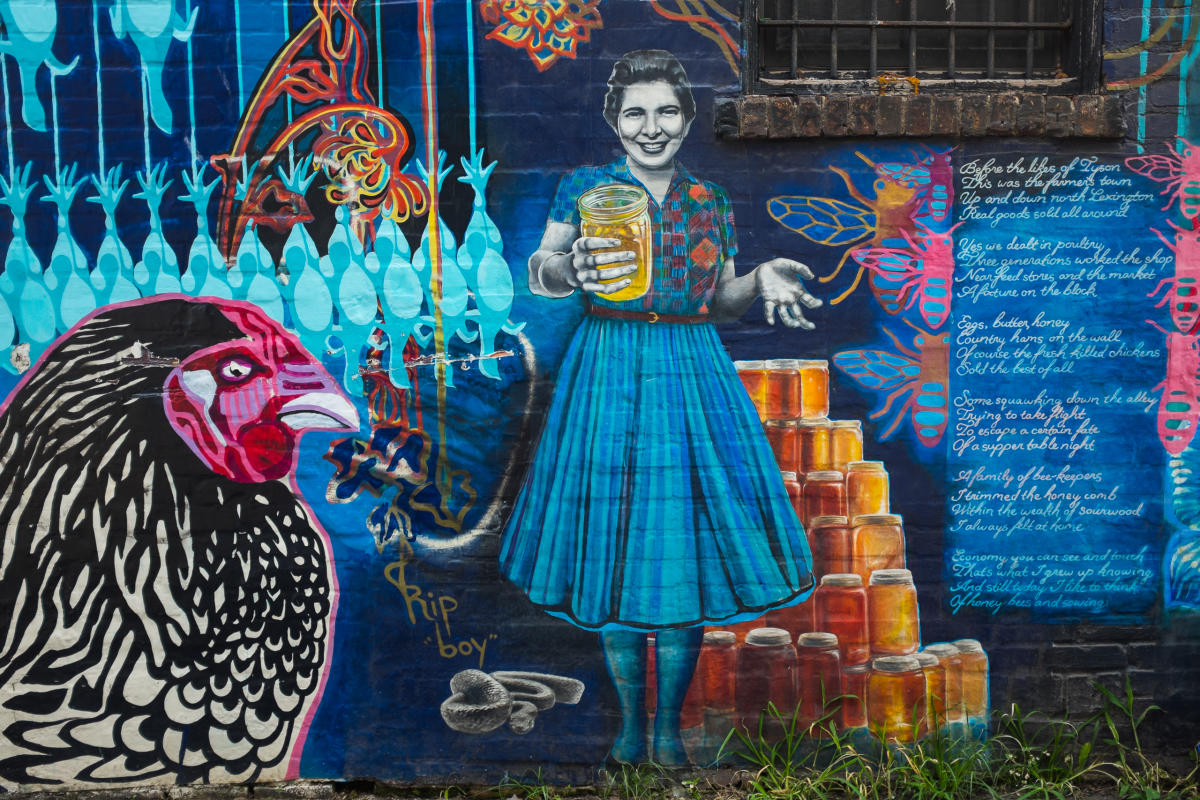The mural depicted on the side of the building is a rich and vibrant scene filled with various elements that highlight a mix of agriculture and historical life. Central to the mural is a smiling woman with short, dark hair clad in a blue short-sleeved dress, cinched at the waist with a thin brown belt. She is holding a jar of honey in her right hand and presenting it toward the viewer in a welcoming gesture. Surrounding her, especially on the right side, are numerous jars of honey stacked in a pyramid shape. 

To the left of the woman, painted prominently on the wall, is a large black and white chicken with a red face and white beak. Not far below, a snake appears with the words "R.I.P. boy" written over it, and nearby, dead chickens hang from ropes in the top left corner. The mural features vibrant colors such as reds, blues, pinks, purples, black, grayish white, oranges, and yellows, bringing the entire scene to life.

Additionally, there's detailed text written in white cursive, conveying a historical narrative about the local trade in poultry, honey, and other goods, possibly indicating ties to Tucson and North Lexington. Alongside the rich textual history, a window with bars can be seen at the top right corner of the mural, adding to the authenticity and depth of the scene. Grass painted at the base of the mural completes the rustic, lively depiction. The overall atmosphere suggests a thoughtful homage to local heritage, possibly hinting at a connection to a restaurant or market.